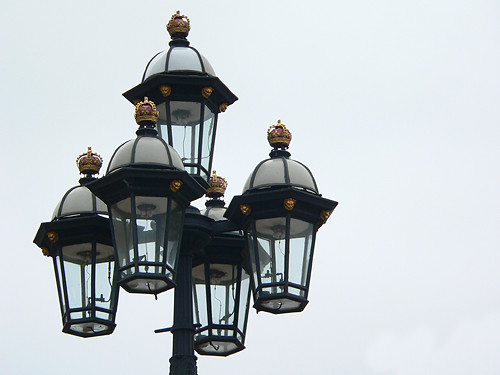The image showcases a tall, ornate streetlamp designed to emulate the old-fashioned gas lamps of the late 1800s to early 1900s, although it is clearly modern and likely electric. The lamp features a hexagonal glass base encased in black slats, topped by a platform resembling a canister lid. A striking dome with black and white stripes sits above this base, crowned by an exquisite gold filigree emblem. The main lamp is surrounded by four smaller lamps, symmetrically arranged at about halfway down the central pole, each mirroring the intricate design of the primary lamp. The entire structure stands against a backdrop of a bluish-gray sky, making the ornate details and gold fixtures stand out vividly.